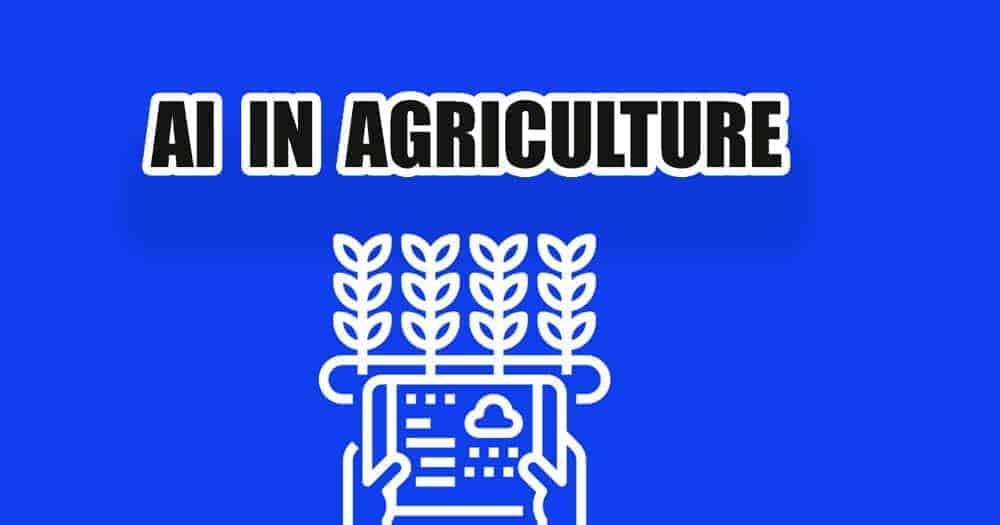The image features a bright blue background with bold, black block lettering outlined in white that reads "AI in Agriculture." Below the text is a white graphic depicting two hands holding a tablet. Emerging from the tablet are four plant-like designs, suggesting crops such as wheat or corn. The tablet itself is detailed with a small cloud icon in the top right corner and three square buttons in the top left corner. Additionally, the tablet displays five horizontal lines and six smaller squares in the bottom right corner.